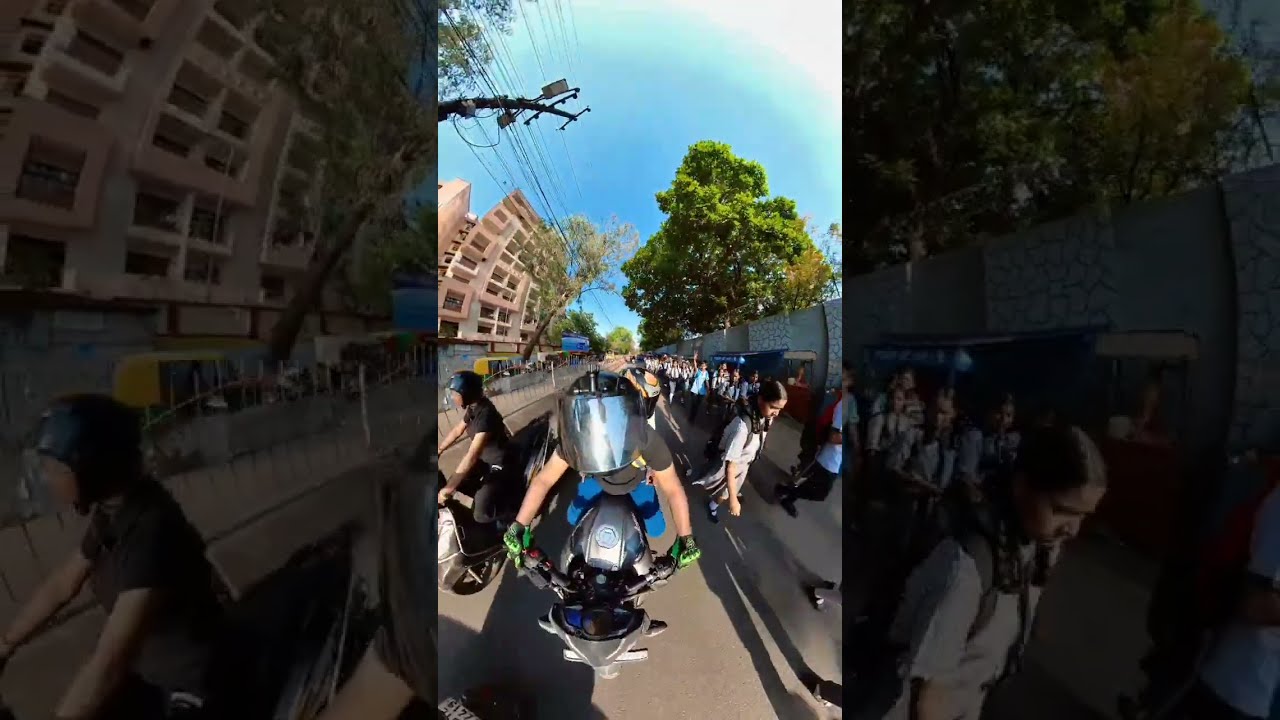The image is a color photograph captured with a fisheye GoPro lens, giving it a distinct wide-angle, slightly distorted view. It depicts a lively street scene in an urban area, where multiple pedestrians walk along an asphalt road. A focal point in the center shows two individuals riding European-style scooters, both donned in helmets with visors. One rider is identifiable by a black short-sleeved shirt and green gloves. The scene is bustling with bystanders, some possibly cheering on as if witnessing a casual race or an organized event. In the backdrop, a tall apartment complex with visible balconies stands against a sunny, blue sky with occasional clouds. Several elements like a gray concrete and stone wall, a green leafy tree, and another smaller tree with sparse foliage add to the scenic details. Overhead, power lines or possibly tram wires stretch across, enhancing the urban vibe. The photograph, with its high-angle shot, encapsulates a vibrant day outdoors filled with communal activity.